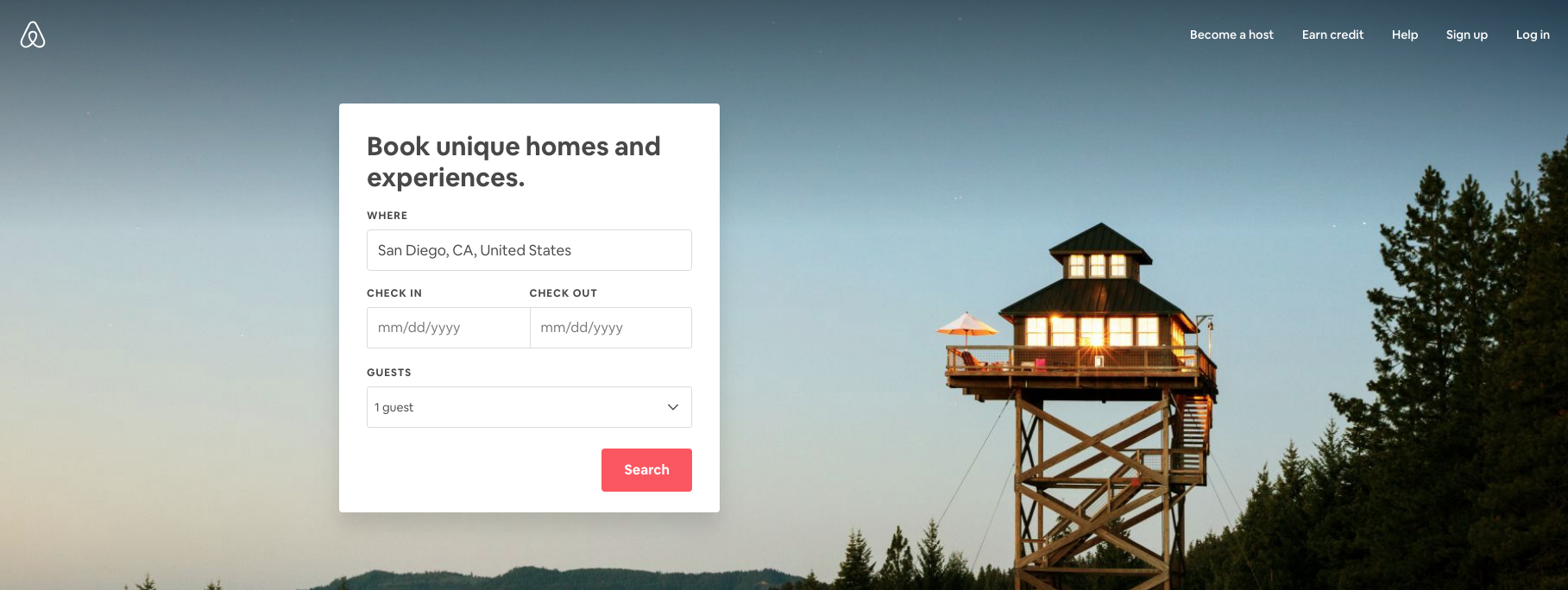The image appears to be a screenshot of the Airbnb homepage, featuring a picturesque sunset scene as the background. The evening sky is filled with warm hues, suggesting the sun is setting. To the right and bottom right of the image, there are trees, adding a touch of nature to the scene. Dominating the right side is a charming wooden tower with a small house perched at the top, adorned with an umbrella on its deck. Lights within the house create a cozy and inviting ambiance.

On the left side of the image, a pop-up box invites users to "Book unique homes and experiences." In this box, "San Diego, California, United States" has been entered as the desired destination. Below that, fields for check-in and check-out dates are available for user input. A drop-down menu shows one guest is selected for the stay. At the bottom right of this pop-up box, there is a prominent red button labeled "Search."

In the top right corner of the image, several options are available: "Become a Host," "Earn Credit," "Help," "Sign Up," and "Log In," offering users a range of actions to enhance their Airbnb experience.